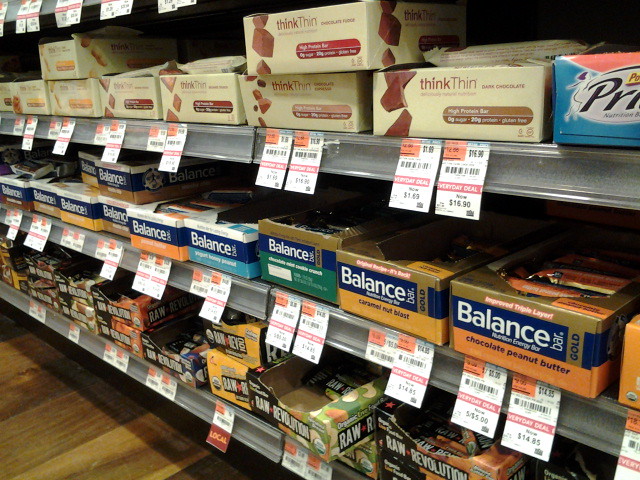This photograph showcases a shelf stocked with a variety of nutrition and diet bars, prominently featuring brands such as ThinkThin and Balance Bar in diverse flavors. The ThinkThin bars are displayed in tan packaging adorned with reddish font, while the Balance Bars have an eye-catching design of gold, blue, and white with different colors distinguishing various flavors. Visible on the shelves are price tags in red, white, and black, adding to the retail ambiance. Below the shelving unit, there is a glimpse of a mid-toned, blonde-leaning wood floor, with soft shadows cast across its surface, providing a warm and inviting backdrop.